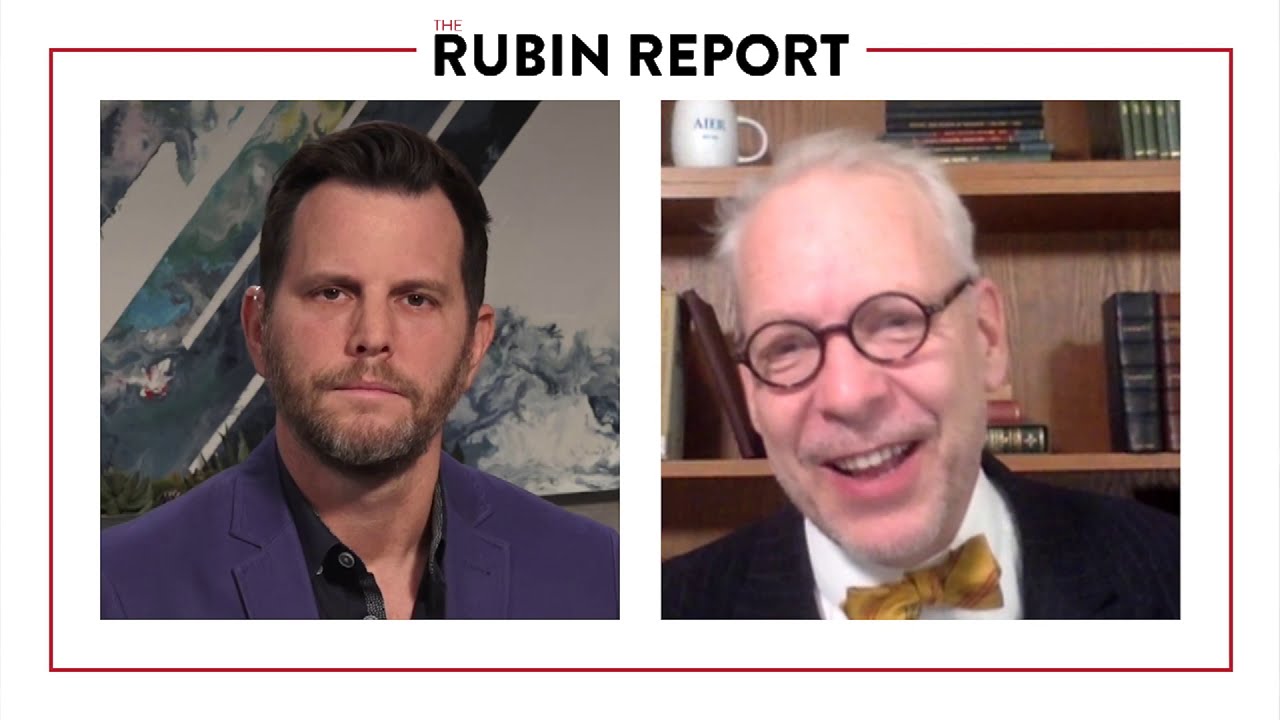The image is a split-screen of a news broadcast titled "THE RUBIN REPORT," with the title in bold black letters except for "THE," which is tiny and in red. A red rectangular border surrounds the two separate video feeds. On the left, a man with short brown hair and a scruffy beard wears a purple suit jacket over an unbuttoned dark blue shirt, against a backdrop of swirling greenish-blue and yellow diagonal stripes, and what seems to be a small patch of grass. He appears a bit confused or angry. On the right, an older man with white hair and a receding hairline is smiling. He has circular glasses and wears a black blazer, white shirt, and gold bow tie. Behind him is a neat bookshelf filled with old books and a white coffee mug. Both men are likely participating in a discussion on "THE RUBIN REPORT."